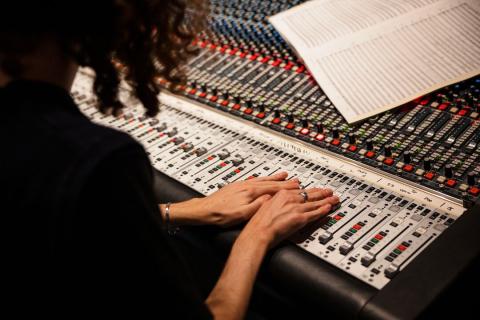This photo, rectangular and wider than it is tall, captures an over-the-shoulder perspective of a woman working in an industrial-style music studio. The focus is on her hands positioned on a professional soundboard filled with numerous buttons and controls. She is wearing a black long-sleeve shirt, a silver bracelet on her right wrist, and a ring on her middle finger. Her unmanicured hands delicately adjust the soundboard settings. Her curly, brown hair slightly obscures her face, blurring into the background. Above the soundboard, there is a piece of white paper with black writing, possibly sheet music or notes, adding to the sense of a recording studio environment.